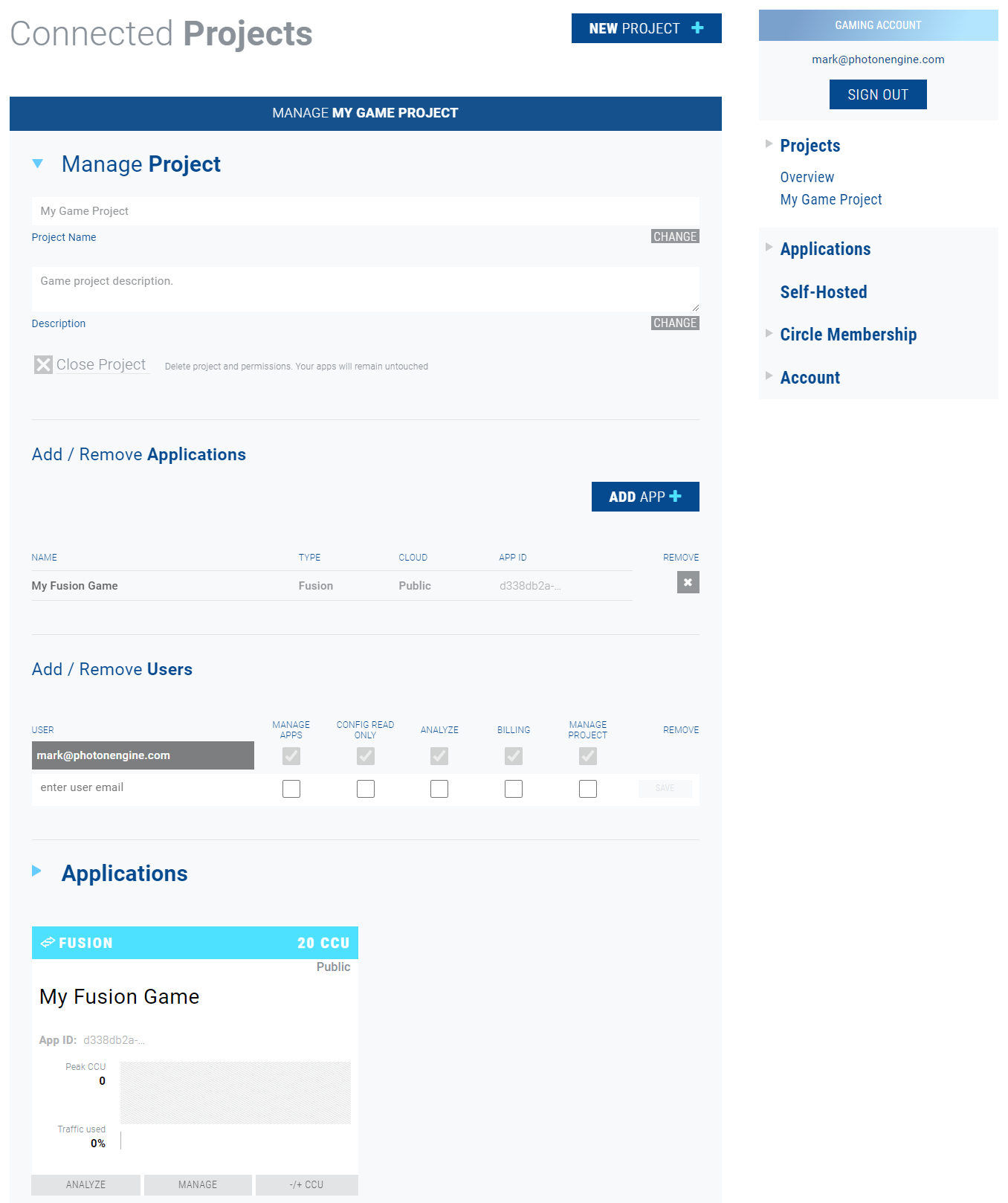Here is a well-organized, detailed caption for the described image:

---

The image depicts a web interface with a clean, white background. In the upper left corner, there is gray text that reads "Connected," and just below it in a slightly darker font, the word "Projects." On the right side of the header, there is a blue button labeled "New Project" with a plus symbol. The word "New" is displayed in a darker white, while "Project" is in gray and the plus symbol is in light blue.

To the right, there is a text box with a gradient background that transitions from dark blue on the left to light blue on the right. Within this box, the words "Gaming Account" are written in white. Below it is an email address, followed by a blue "Sign Out" button with white text. On the same vertical line, a navigation menu lists the following items: "Project Overview," "My Game Project," "Application," "Self Hosted," "Circle Membership," and "Account."

On the left side, a dark blue tab reads "Manage My Game Project." Below it, on a gray background, there is an input area labeled "Manage Project" where users can type in project specifics. This section includes options such as "Manage Project," "Game Project," "Remove Ad Applications," and an "Add App" icon on the right. Further down, the interface displays "My Game Fusion," "Fusion Public," and an "ID Code" next to functionalities like "Remove," "Add," "Remove Users," and "User." Another gray box with white text shows an email: "mark@photonengine.com," indicating the user has access to manage apps, configure read-only settings, analyze billing, and manage the project.

Additionally, there is another input field for entering an email address. Below it, under applications, "Fusion 20cc" is displayed on a light blue background with blue text, along with "My Fusion Game." At the bottom left, there is a blank gray space.

---

This cleaned-up and organized caption provides a comprehensive description of the web interface elements.